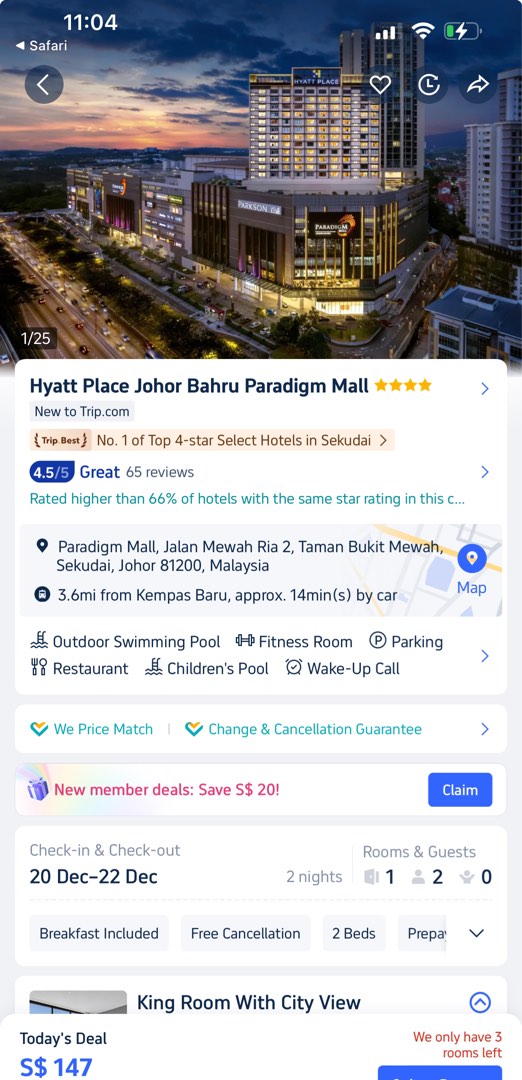This image is a screenshot of a smartphone displaying information about the Hyatt Place Johor Bahru, located near the Paradigm Mall. At the top of the screen, the time is shown as 11:04 AM on the top left, and a charging battery icon with a lightning bolt is visible on the top right. Below these icons, there are navigation and action buttons, including a back button on the top left and a heart icon, a clock symbol (presumably for refreshing), and a share button on the top right.

The main content features an image of the exterior of the Paradigm Mall, emphasizing the connection to Hyatt Place Johor Bahru. This hotel is rated 4 out of 5 stars based on 65 reviews, achieving an overall score of 4.5 out of 5, which is labeled as "Great." The green text indicates that it is rated higher than 66% of other hotels with the same star rating in the Sekudai area. Additionally, it is highlighted as the number one choice among the top four-star hotels in Sekudai. The bottom section displays the booking website, newtotrip.com, which provides the detailed review summary.